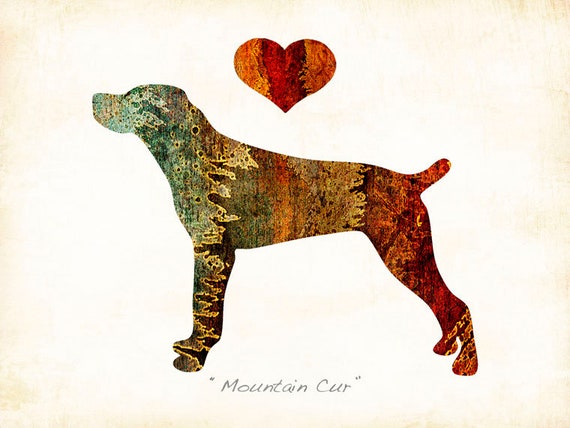This digital artwork features a detailed, side-view silhouette of a dog placed centrally on a white background. The dog and the heart above it are adorned with a marbleized texture that transitions through various colors, creating a rainbow-like effect. The dog's silhouette begins with a greenish hue around the head, moving into shades of red, brown, and orange, with notable elements such as tan sections and even lace-like patterns. The dog is designed in a collage style, incorporating intricate designs like circles, splotches, stripes, and wood-like textures, with some areas resembling realistic elements such as trees. The heart above the dog's head, which matches the marbleized look, features hues of yellow, orange, and red. Below the dog, there is handwritten text that reads "Mountain Cur."